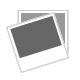The image is a collage of four square panels detailing the features of a pair of leather shoes. The top left panel showcases a close-up of the front of the shoe, highlighting its neat stitching with the text "Neat Stitching." The top right panel focuses on the upper part of the shoe, emphasizing its alligator hornback leather texture with the text "Alligator Hornback Leather." This panel specifically highlights the characteristic ridges found in alligator skin. The bottom left panel shows the interior of the shoe from a top angle, described as having a breathable lining, which appears to be a light tan or greenish-brown color, adding a sense of comfort. Lastly, the bottom right panel displays the anti-skid sole of the shoe, presenting the textured areas on the sole designed to provide grip and prevent slipping, with the text "Anti-Skid Sole." The central text of the image simply states "Details," tying all the featured aspects together.